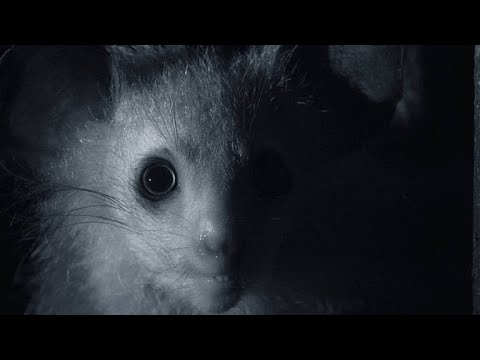This is a black and white (or bluish gray and white) photo of a creature with an eerie and unsettling presence. The animal, resembling a rodent with human-like features, is looking directly at the camera with wide, beady eyes that have fully dilated pupils, giving it a creepy, almost mutant-like appearance. The dim lighting casts shadows across the left side of its face, highlighting the large, rounded ears and the partially open mouth with visible teeth, while the right side fades into darkness. The creature's face, with its peculiar human-like nose and mouth, adds to the haunting atmosphere of the image, making it appear as if captured candidly from a horror show.